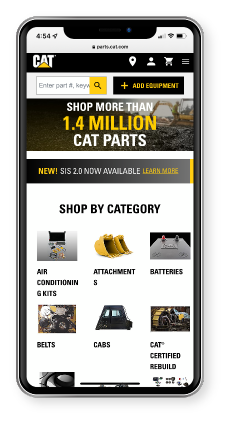This is a detailed screenshot of an iPhone home screen taken at 4:54, featuring a variety of on-screen elements pertinent to the user interface of the Cat brand's mobile application. The status bar indicates that location services are active, the device is connected to Wi-Fi, and the battery is approximately 60% charged, with two bars of cellular service. 

Central to the image is the Cat app interface, distinguished by white text featuring the iconic yellow triangle logo. The top of the screen features a yellow button with a magnifying glass icon inside a search bar, flanked by three icons: a location pin, a user profile button, and a shopping cart. Below this interface, a black rectangular button marked "Add Equipment" in white text with a yellow plus sign is prominently displayed.

A highlighted banner backdrop features a photograph of a large crane and includes the promotional message “NEW CIS 2.0 NOW AVAILABLE” in yellow text on a black background, supplemented by a “Learn More” call to action also in yellow. Beneath this banner lies a shopping section headlined with "Shop More Than 1.4 Million Cat Parts," followed by product categories such as "Air Conditioning and Kits," suggesting a well-organized and comprehensive parts inventory.